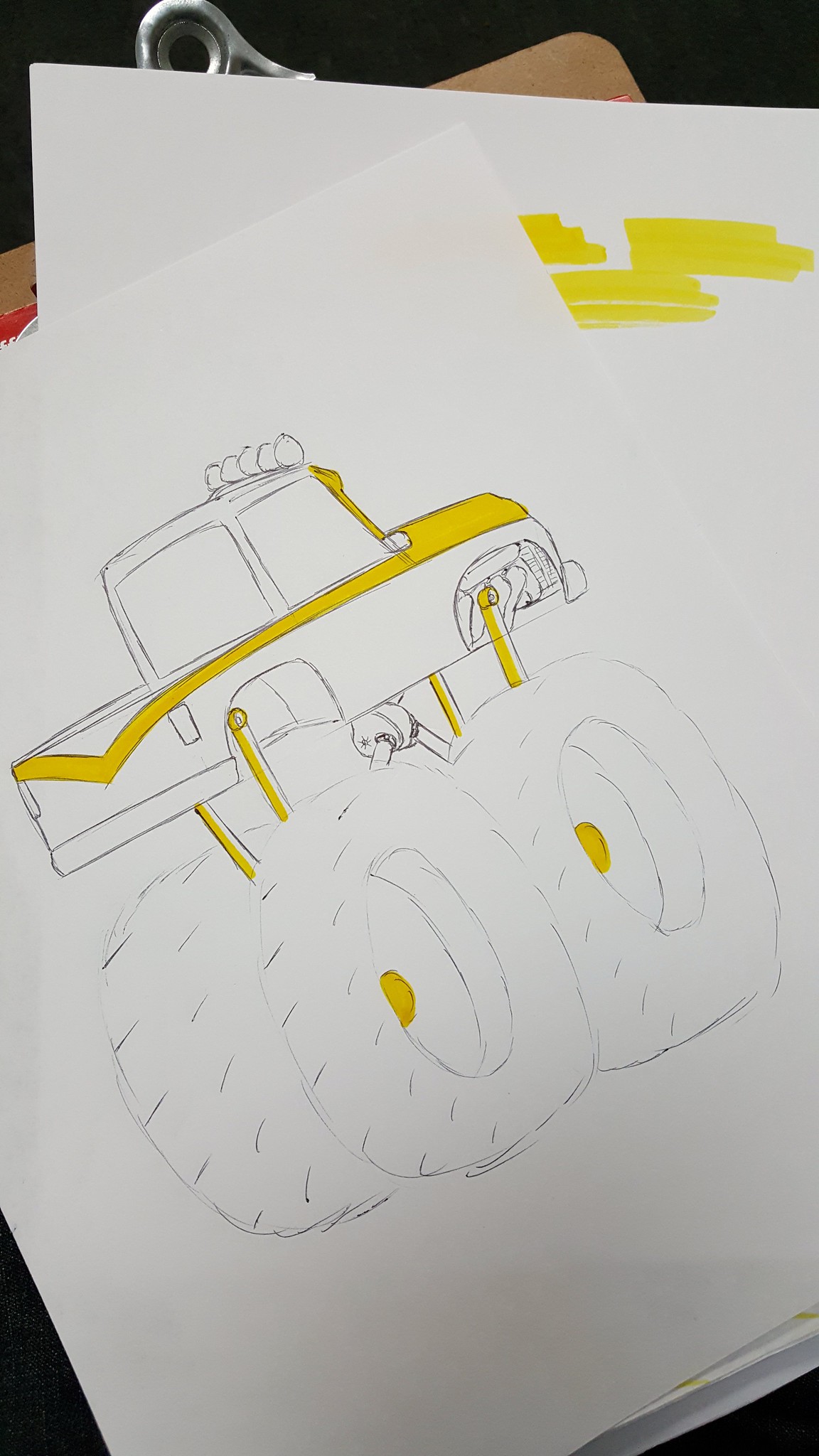This vertically cropped color photograph showcases two pieces of white copy paper placed on a clipboard. The top sheet, lying diagonally, features a detailed pencil drawing of a monster truck. The drawing is accentuated with yellow highlights on various parts of the truck's body. The truck is depicted with large, circular tires, also highlighted in yellow, connected to a stick-like mechanism that extends from the body of the truck. A hydraulic system detailed beneath the chassis, between the wheels, adds a sense of mechanical realism to the illustration. Additional small circles atop the truck represent lights. Visible on the blank sheet below are smudges of yellow marker, likely indicating attempts to ensure the marker was functioning properly before use.